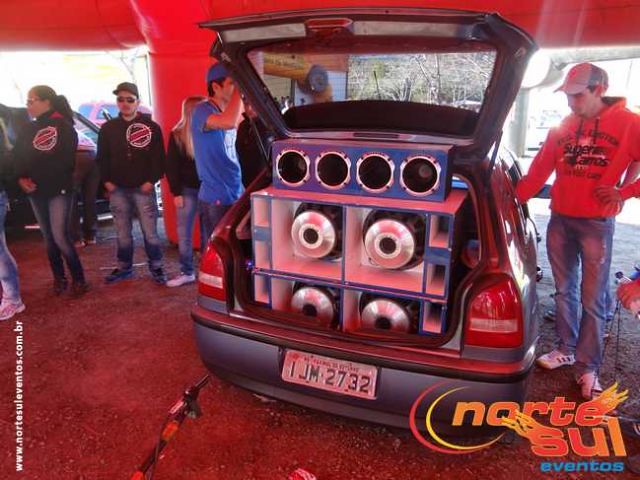In a spacious garage with a red roof and a gravel floor, a meticulously modified 1978 Chevy Hatchback with the license plate IJM2732 showcases an extraordinary sound system. The back of the car features four large blue speakers with white cones, topped by another panel containing four subwoofers, making for a striking sound setup. Various people are gathered around the car: to the far left, two individuals in jeans and black hoodies, a man in a blue shirt placing his hand on the car's open hatch, and a blonde person standing behind him. On the right, a man in a red hoodie, white cap, jeans, and white sneakers has his arm through the back window. This scene is associated with Norte Sul Eventos, as indicated by distinctive branding in the bottom right-hand corner of the image, suggesting that the event might be in Brazil.